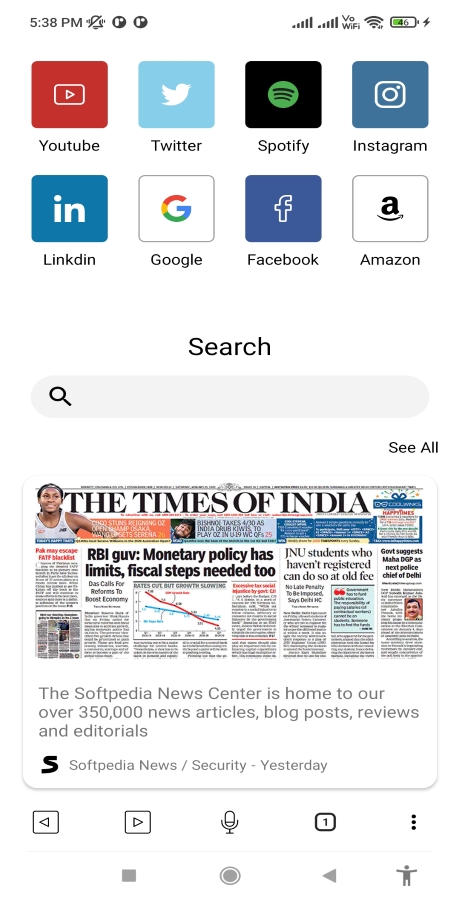This is a detailed phone screen capture of a search page primarily dedicated to news. The screen is divided into three main sections. 

In the upper section, there are two rows, each containing four icons representing popular applications. The first row features YouTube, Twitter, Spotify, and Instagram. The second row includes LinkedIn, Google, Facebook, and Amazon.

Centered on the screen is the search box, which is currently empty. Directly below this search box, there is an image link to the Times of India newspaper front page. The image is captioned with the text: "The Softpedia News Center is home to over 350,000 news articles, blog posts, reviews, and editorials."

At the very top of the screen, the time is displayed as 5:38 PM, alongside icons indicating the current signal strength, Wi-Fi signal, and battery level, which is at 46%.

At the bottom of the screen, there are navigation icons, including a back button, a forward button, a microphone button for voice input, and a button indicating recent notifications.